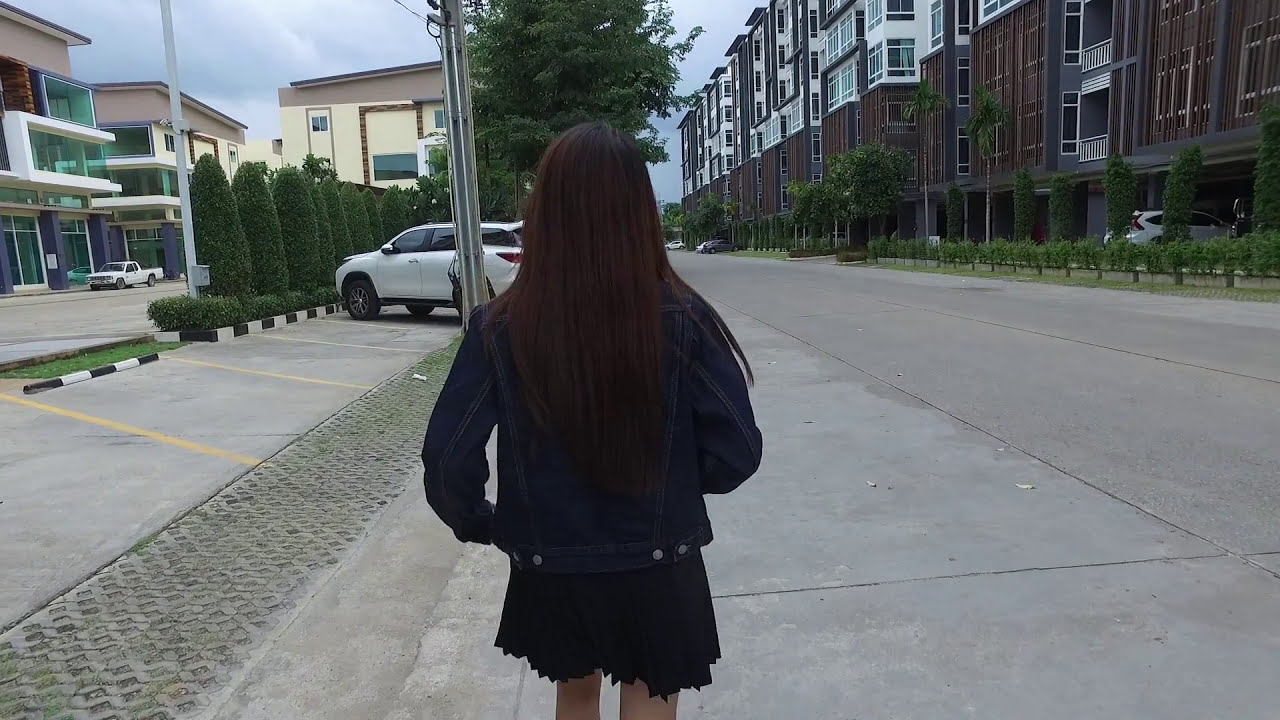In the foreground of the image, a young woman with long brunette hair walks away from the camera, her back to the viewer. She wears a dark blue denim jacket and a short black skirt, exposing her left thigh and the upper part of her right leg. The street she's on merges indistinctly with what appears to be a sidewalk or side path, devoid of any boundary. To her left, yellow markings delineate parking spaces, where a white SUV is parked. Further to the left, a brown and white building, possibly housing, is partially obscured by a line of small trees. In the background, a cluster of buildings with various hues—brown, white, and yellow—stand alongside the street, many with numerous windows. Along the right side of the image, another white vehicle and a darker car are parked further down the road. Additional greenery, including small and slightly larger trees, lines the street on both sides. The woman looks down the street, bordered by parked vehicles and buildings, which extends from the bottom of the image toward the horizon.